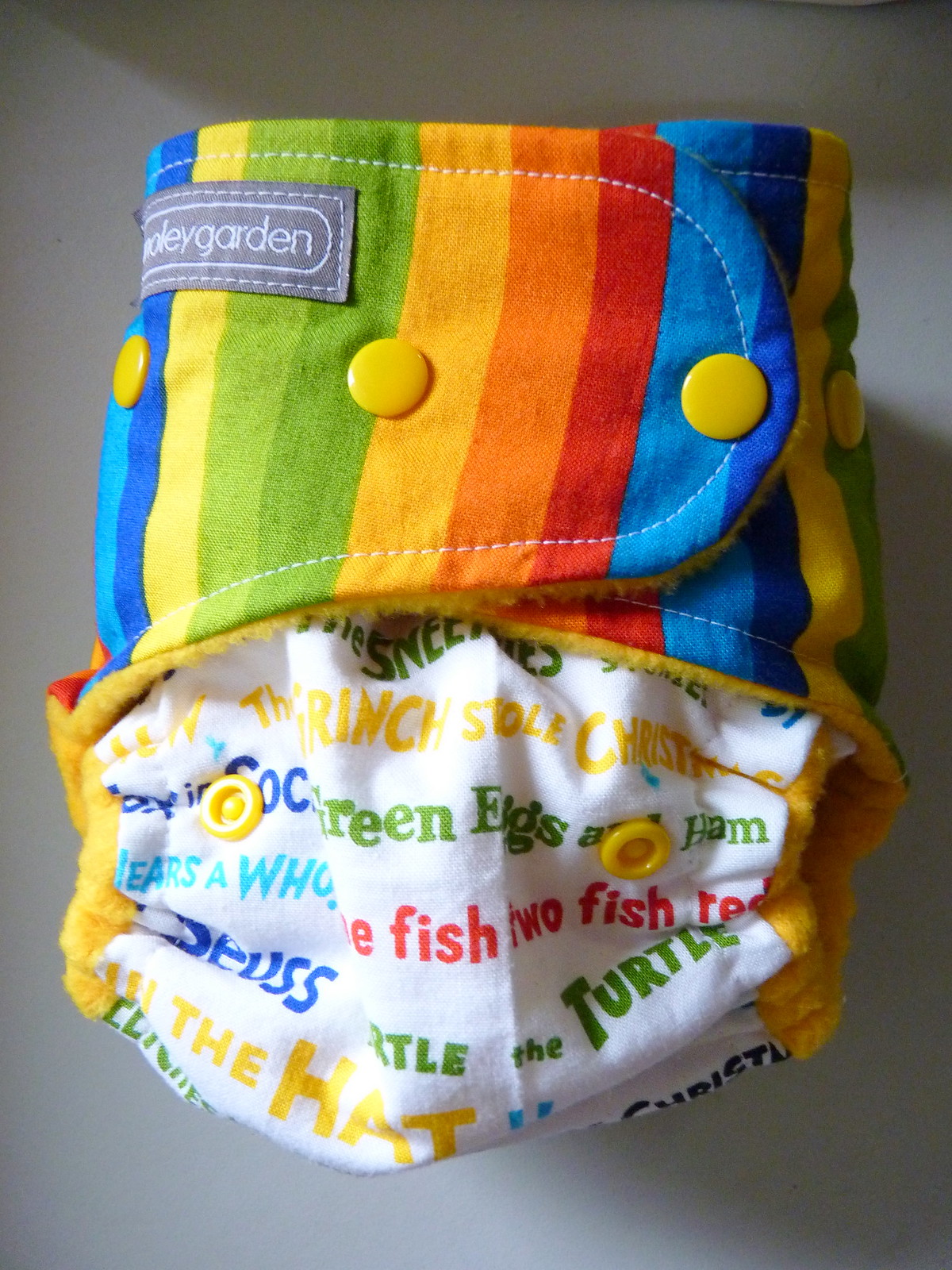This close-up photograph features a cloth baby diaper with a colorful rainbow pattern at the top. The vibrant stripes include light blue, dark blue, yellow, light green, green, orange, and red, and are complemented by yellow snap buttons. On the top left, there's a gray tag with white text that reads "Poli Garden." The lower half of the diaper is white and includes multicolored text with playful phrases such as "green eggs and ham," "one fish, two fish," and "turtle." The object appears to be laying on its side, possibly on a table or a photo backdrop.